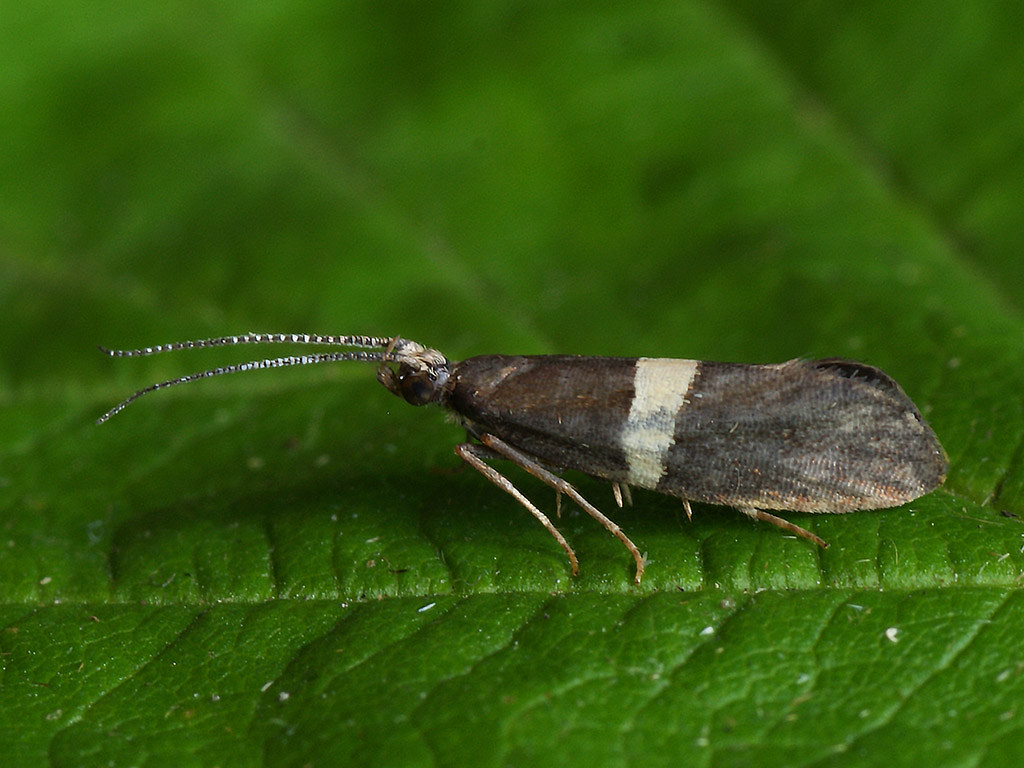In this detailed close-up image, we observe a sizable insect resting on a vibrant green leaf. The leaf's texture is clearly visible, with fine grains, lines, and even specks of dust, as though viewed through a magnifying glass. The insect, which appears to be a cicada, has a distinct body shape that is dark brown with a prominent horizontal white stripe across its midsection, giving the appearance of a deliberate paintstroke. The insect's six legs, three of which are clearly visible, support it on the leaf. It has an elongated, teardrop-shaped body and a disproportionately small head. The bug's large, shiny eyes and long antennae, which are black with tiny white stripes, are striking features. The antennae extend outwards, almost as long as the insect's body. The overall scene portrays the insect as if it's patiently waiting on the leaf, possibly preparing to feed.